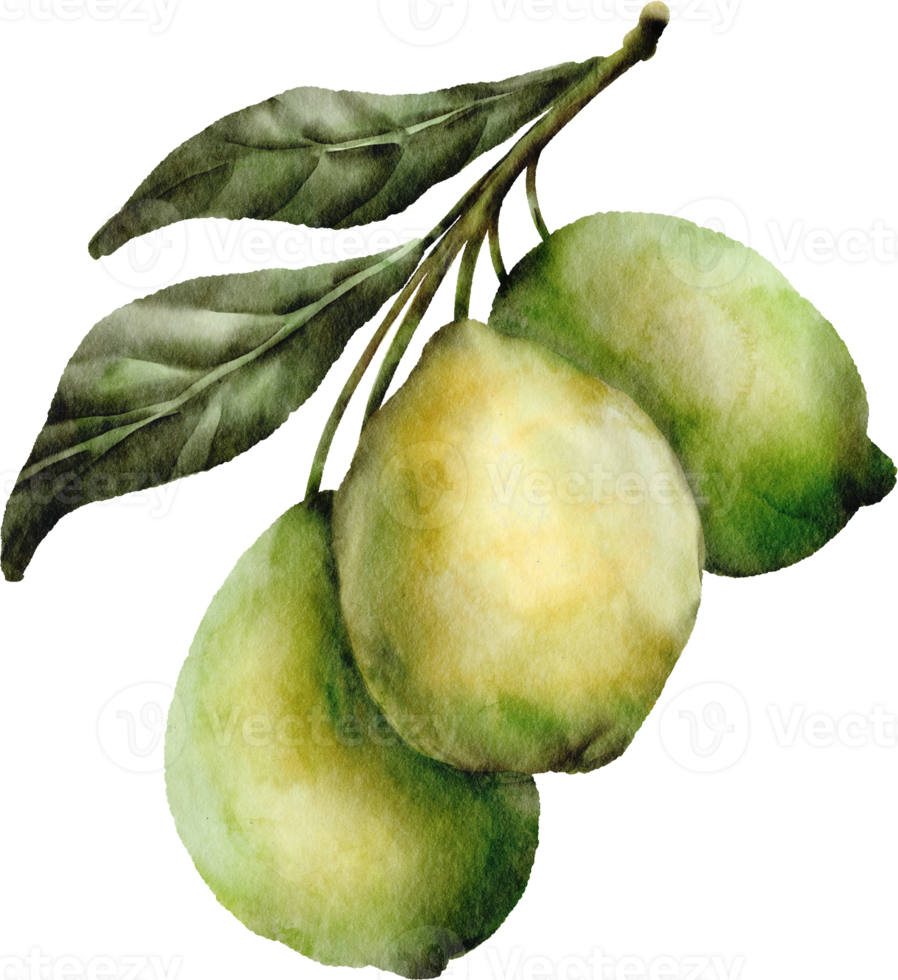This image is a watercolor painting depicting three pears hanging from a branch. The pears vary in shades of green, indicating different stages of ripeness, and each pear has small protrusions at their ends. Accompanying the pears are two green leaves, all set against a white background. Embedded within the artwork is a subtle, see-through watermark composed of the word "Vecteezy" repeated throughout in fine print, which suggests that the image is sourced from the Vecteezy platform. The overall composition appears delicate and detailed, highlighting the texture and nuances of the pears and leaves vividly.